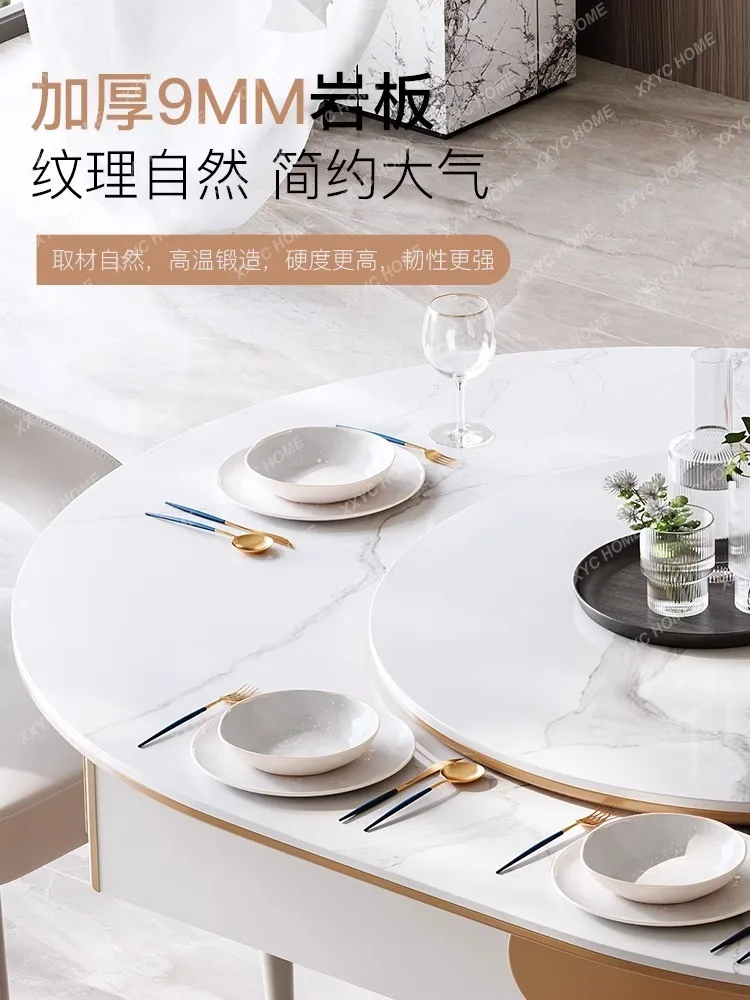The image depicts a sophisticated table setting on a contemporary marble-like white table. At the center of the table is a large, marbleized Lazy Susan, adorned with a shallow metal platter holding a clear glass vase with small flowers immersed in water. The table appears to be set for a dining occasion with three place settings along the left side, each featuring white plates and bowls, as well as unique cutlery with black handles and gold-toned ends. Notably, there is one wine glass at the head of the table, hinting it might be reserved for an adult, possibly suggesting a family setting. The scene hints at an Asian or Japanese ambiance, supported by foreign writing, including Chinese characters and the number "9MM" integrated into the text, suggesting the image could be part of an advertisement for an Asian restaurant. Additional furnishings, like a possible bench and other dishes, are subtly visible in the background, enhancing the modern and elegant atmosphere.